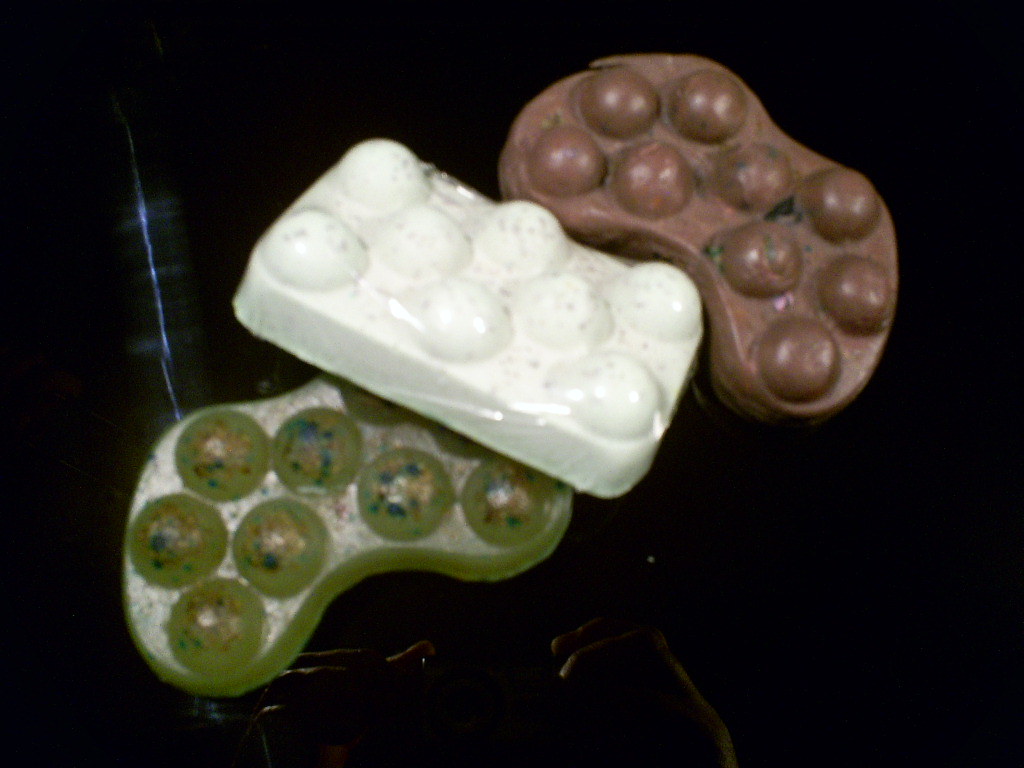The image features three distinct candies against a predominantly black background, which includes subtle bluish and yellowish reflections. The candies are characterized by a common feature: circular, bump-like designs reminiscent of half-spheres or Lego pieces. The first candy, positioned on the left, is an irregularly shaped green jelly candy. It is somewhat transparent with darker green hues and speckled with colors like blue, yellow, and red. The central candy is a white rectangular piece marked with small reddish-brown spots. The rightmost candy is brown, blob-like, and has spots of yellow, green, and pink. All three candies possess about eight to ten circular bumps on their surfaces. The contrasting backdrop and the intricate candy designs create a visually engaging image.